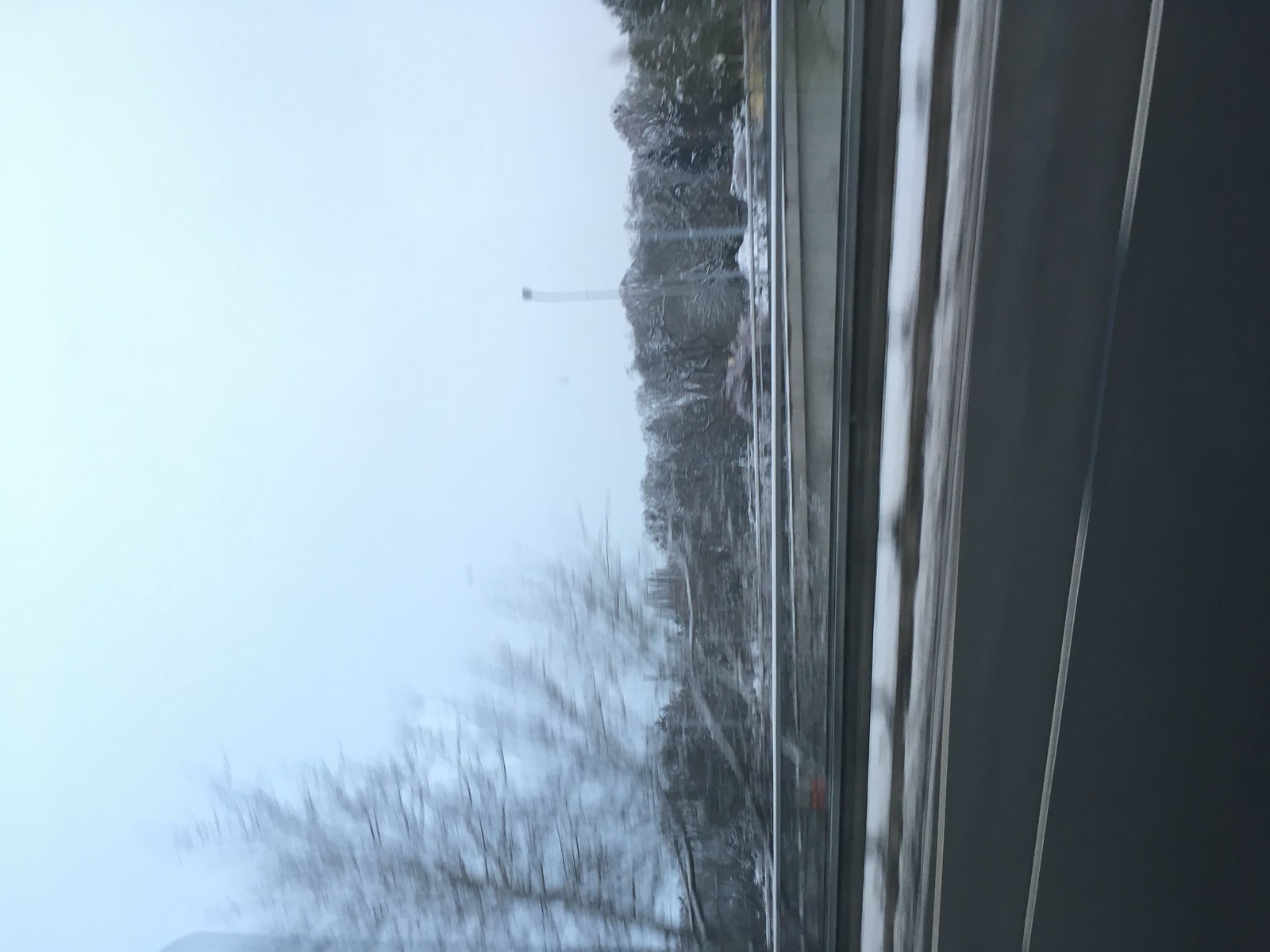This photograph captures a city street scene with black pavement and a light dusting of snow along the roadside. Viewed at an unconventional angle, the street runs vertically along the far right edge of the image, while the sky occupies the left side. This unusual perspective creates an intriguing visual, with a snow-covered area leading into a green grassy tree line, dividing the image diagonally. The tree line, situated horizontally in the center, features tall, leafless trees with bare brown branches stretching upwards to the left. The sky above them is a muted blue, underscored by overcast clouds, enhancing the photograph's unique and striking composition.